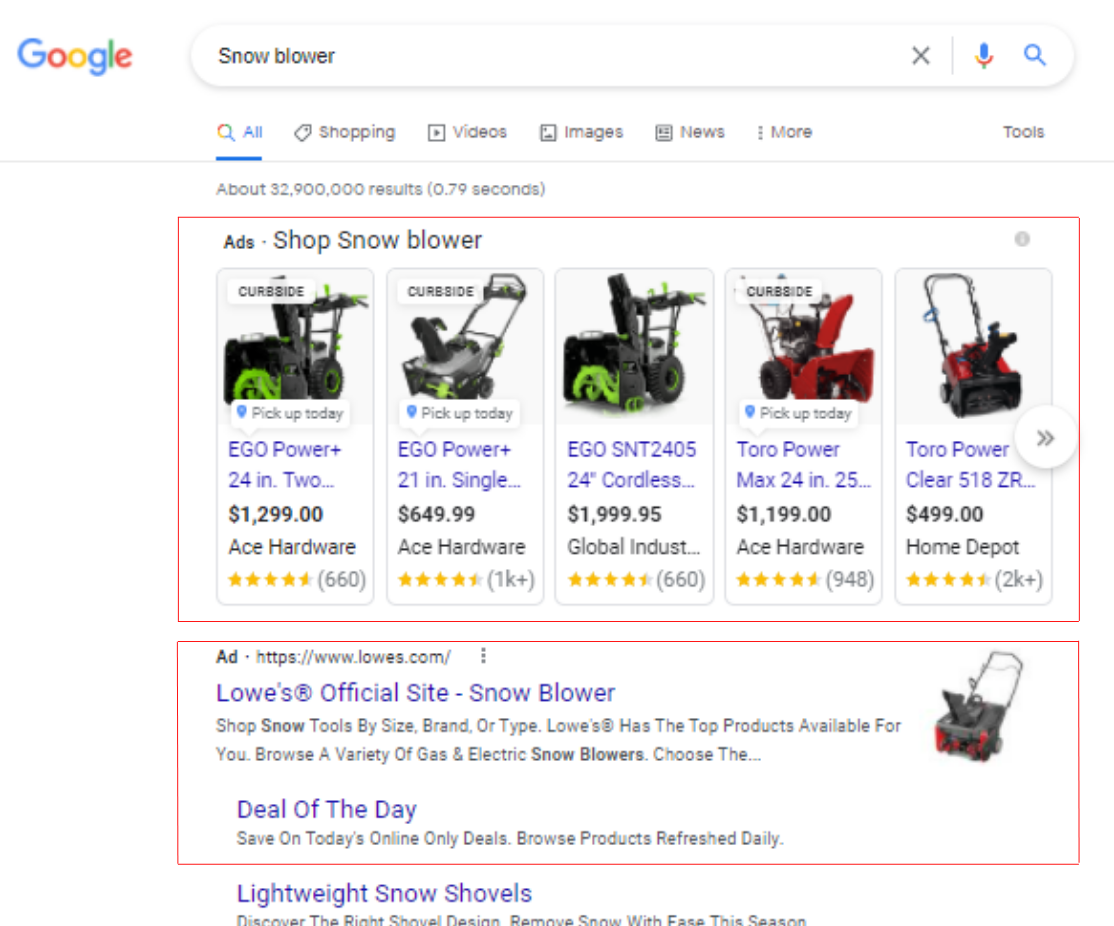This image is a detailed screenshot of a Google search for "snowblower," showcasing two highlighted sections primarily composed of advertisements. The first highlighted section is a collection of shopping ads featuring images of various snowblowers from different retailers. Notable details include:

- Five distinct product ads from retailers such as Ace Hardware (3 ads), Global Industrial (1 ad), and Home Depot (1 ad).
- Two featured snowblower brands: Ego and Toro Power.
- Price range of the advertised snowblowers spans from $499 to $1,999.95.
- Thumbnail images of the products linked to their respective websites invite viewers to explore options further.

The second highlighted section is a text ad located directly below the product images, linking to Lowe's official website section dedicated to snowblowers. It presents:

- A standard promotional image depicting a red and black snowblower.
- The clickable text "Lowe's Official Site: Snowblowers" which indicates a direct link.
- An additional link labeled "Deal of the Day," suggesting special offers.

Below this, an unhighlighted portion of the screenshot mentions "lightweight snow shovels," though it is ambiguous whether this is part of the Lowe's advertising content or an unrelated search result.